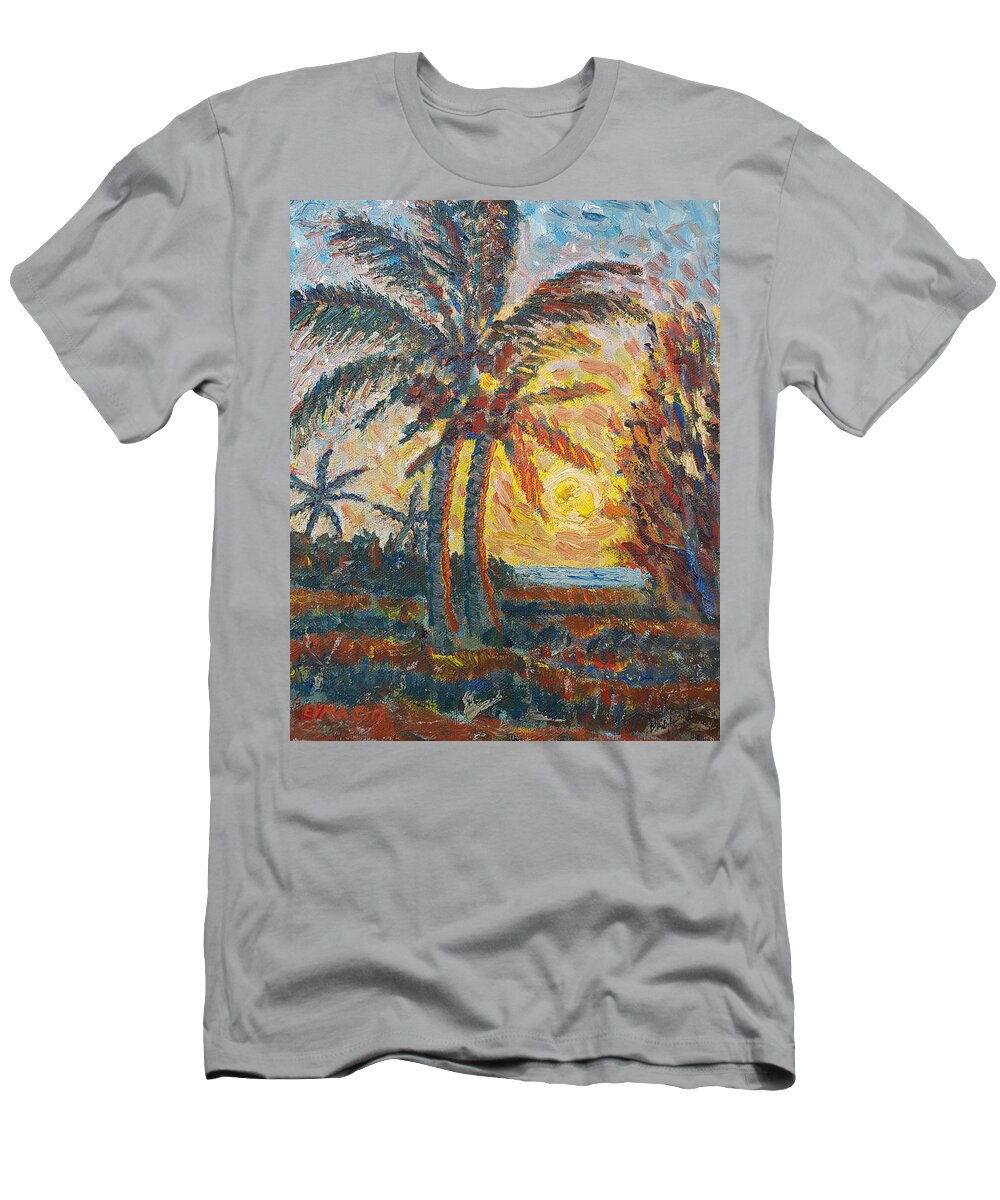This is a detailed color photograph of a slightly wrinkled, soft charcoal grey cotton t-shirt with a round high crew neck and short sleeves, set against a white background. The t-shirt features a large, vertically rectangular screen-printed design on its front, resembling an impressionist painting. This artwork showcases a vivid beach scene with a prominent palm tree in the foreground, adorned with blue and brown hues, possibly indicative of coconuts. There is a secondary, smaller palm tree on the left side of the image, and additional trees or parts of trees are visible in the distant background.

The sky transitions from a deep blue at the top to a vibrant yellow-orange near the horizon, capturing the essence of a sunset or sunrise. Below the palm trees, the ground is depicted with dark brown and blue colors, representing varied vegetation. To the right of the main palm tree, a sliver of sea is visible under the glowing sky. This artwork stands out due to its striking mix of vibrant and deep, dark colors, and large, disjointed brush strokes, giving it a captivating, almost abstract look.